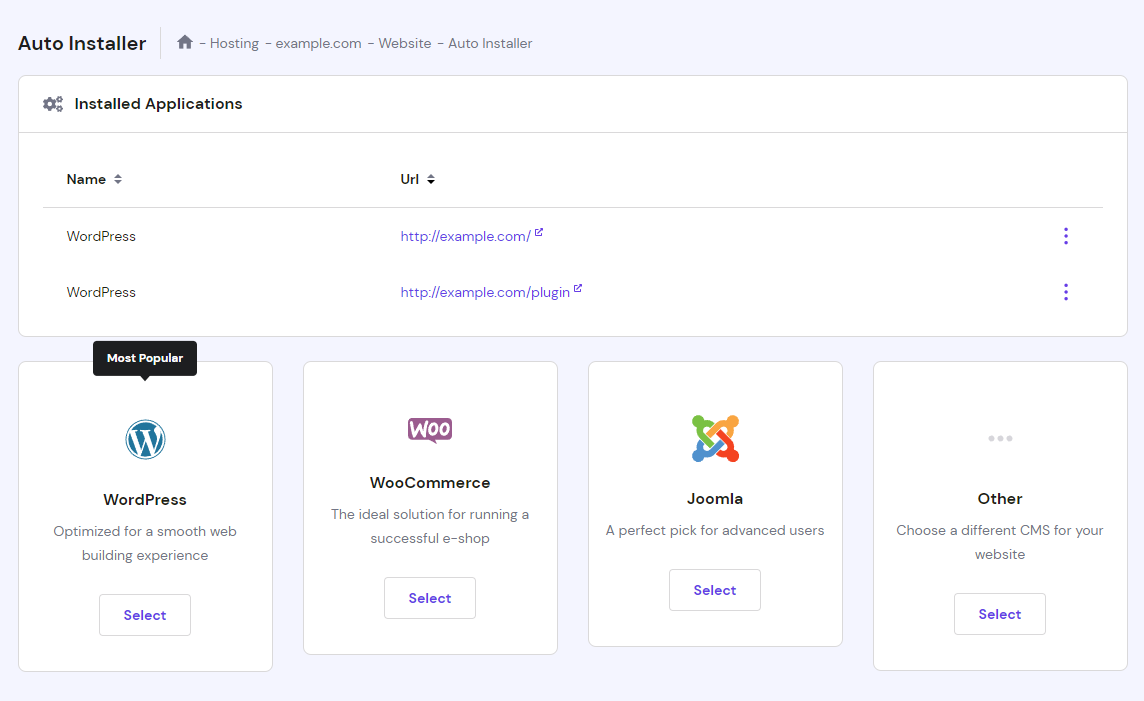The image is a horizontally oriented rectangle with a very pale light blue background. In the top left corner, black bold text reads "Auto Installer," with an unbolded black house icon next to it. Following this, the text reads "Hosting - example.com - Website - Auto Installer."

Beneath that is a horizontally oriented white rectangular section. At the top of this section, bold black text says "Installed Applications," with a settings icon to the left of it. Below this, a fine gray or light blue line separates the section.

Further down, bold black text reads "Name" accompanied by an up and down arrow. To the right of this (though not at the halfway mark of the image) is another text that says "URL," also with an up and down arrow. Underneath this section is another line forming a new box. Inside this box, on the left-hand side, the text indicates "WordPress," and next to it in blue-purple lettering, the URL "http://example.com/...". The second line follows a similar format with "WordPress" and "http://example.com/plugin."

The final section, covering almost the last third of the image, is split into four vertical white rectangular areas on the light blue background. Each area features an icon or logo at the top:

1. **WordPress Logo:**
   - A turquoise box with a white capital "W" and a white border around it.
   - Beneath, bold black text reads "WordPress."
   - Underneath in unbolded black text: "Optimized for a smooth web building experience."
   - A "Select" button in purplish font is centered below.

2. **WooCommerce Logo:**
   - A purple box with white lettering spelling "Woo," inside a horizontal oval.
   - Beneath, bold black text reads "WooCommerce."
   - Below in unbolded black text: "The ideal solution for running a successful e-shop."
   - A centered "Select" button.

3. **Joomla Logo:**
   - Four interlocking links in green, orange, red, and blue.
   - Beneath, bold black text reads "Joomla."
   - Below in unbolded black text: "A perfect pick for advanced users."
   - A centered "Select" button.

4. **Other:**
   - Three horizontal dots where an icon would be.
   - Bold black text reads "Other."
   - Below in unbolded black text: "Choose a different CMS for your website."
   - A centered "Select" button.

This detailed breakdown captures each element and section precisely, offering a clear understanding of the layout and content of the image.